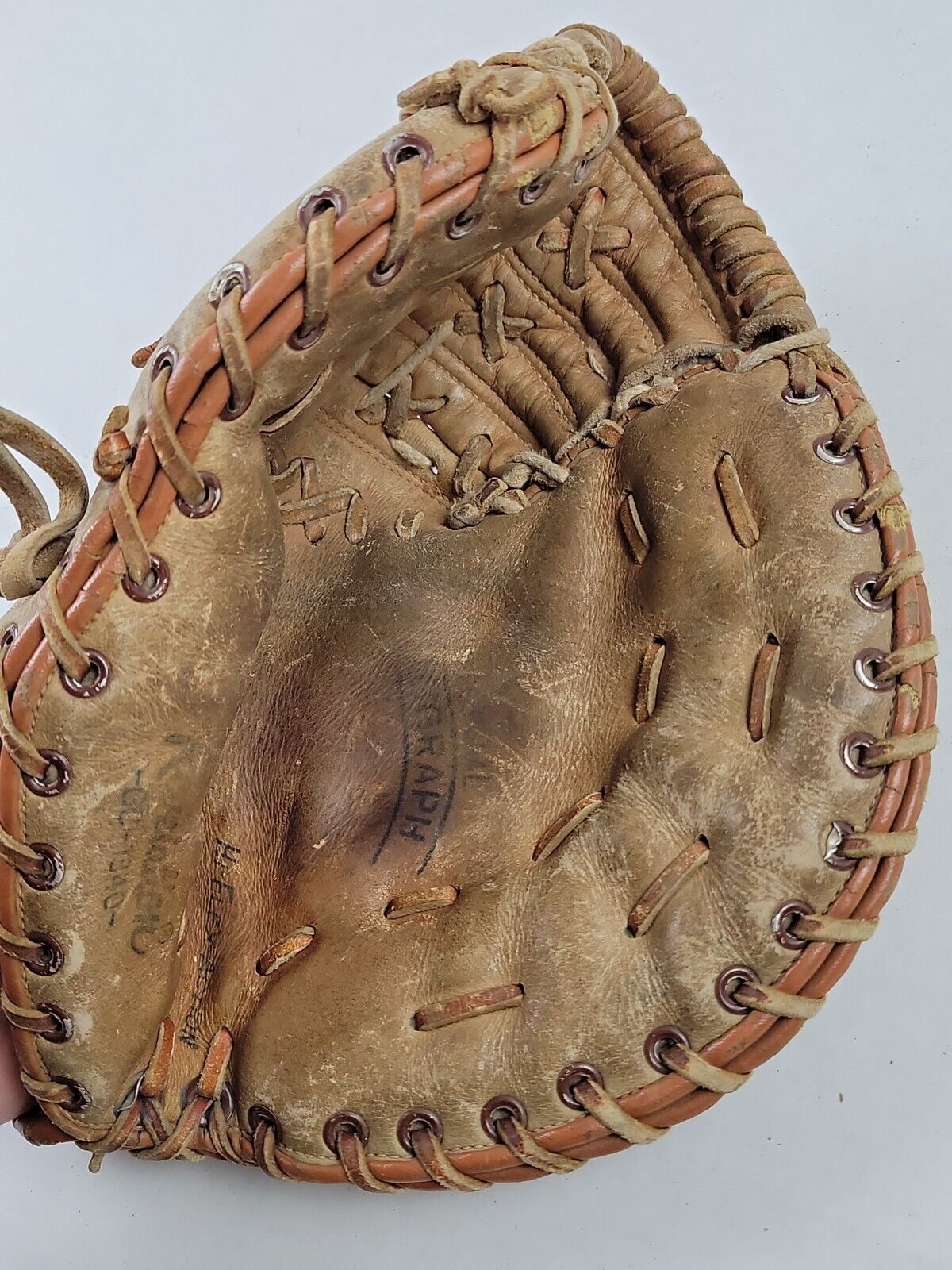This is an image of a well-worn, brown leather catcher's mitt, photographed against a grayish-white background. The mitt, featuring traditional leather stitching and webbing, shows significant signs of use and age, with faded colors, numerous scratch marks, and wear. Handwriting on the mitt is partially legible: "HyFlex action" is clearly stamped, while other inscriptions, like "Revelation GL-1340" and one that might have said "autograph," are heavily worn and difficult to decipher. The glove is designed for a right-handed player, intended to be worn on the left hand. Despite its age, the mitt’s scrapes and fading reveal a history of extensive use and cherishment.